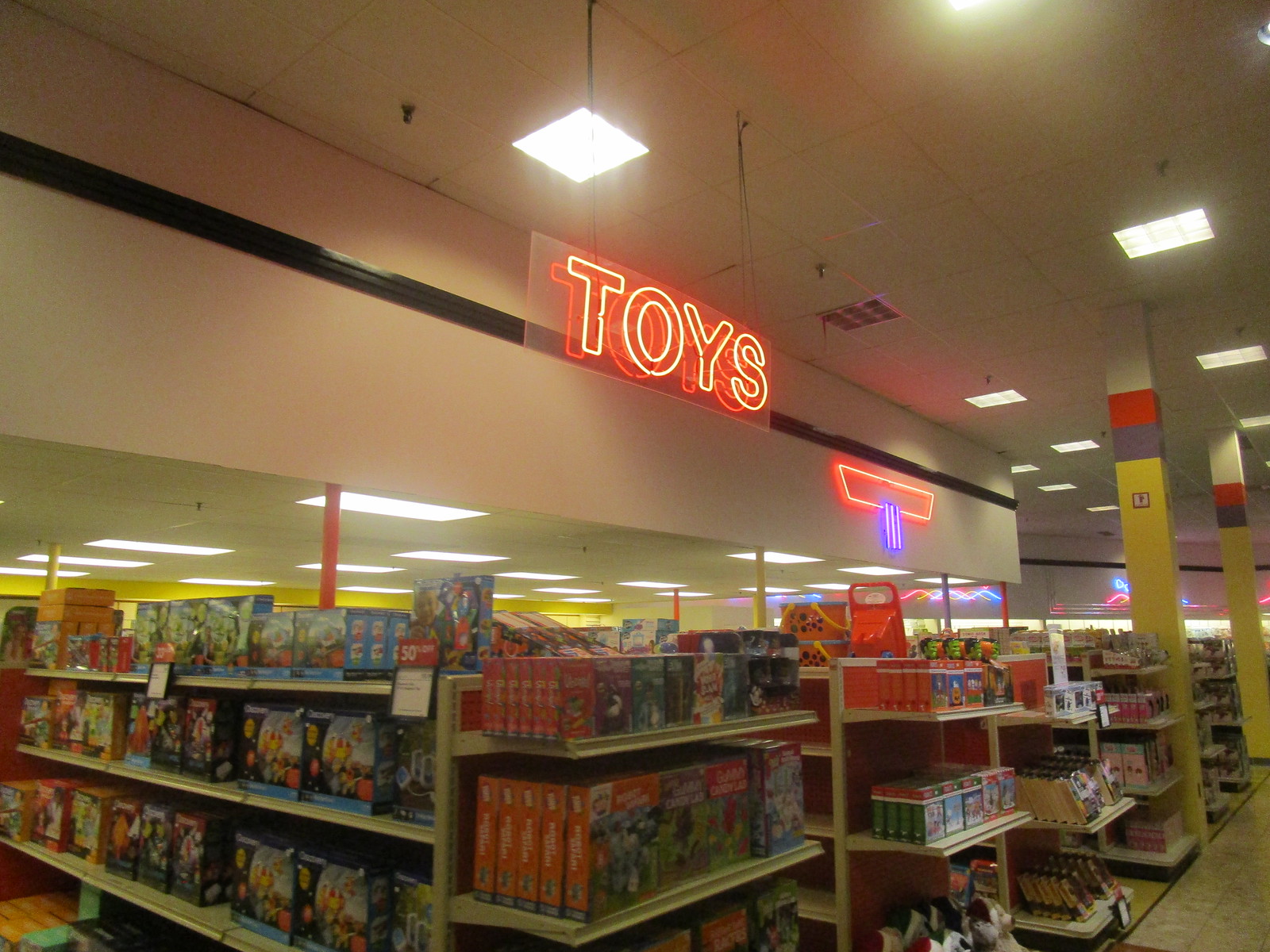This color photograph captures the interior of a toy shop, with an underexposed ceiling giving a darker ambiance to the scene. The ceiling is adorned with both rectangular and square lights, providing a fragmented illumination. Dominating the middle of the photograph is an illuminated sign that reads "toys," bordered by a vibrant red light. Below this sign, several shelves filled with various toys are visible, particularly on the left-hand side of the frame. These shelves are stocked with blue and red boxes, with the central shelves containing a collection of flatter red boxes that might be Lego sets or similar compact items. Towards the right of the photograph, more shelves display an assortment of toy boxes. Tall pillars, painted in yellow at the base and transitioning to blue and red as they approach the ceiling, stand out as structural features and add a splash of color to the scene.